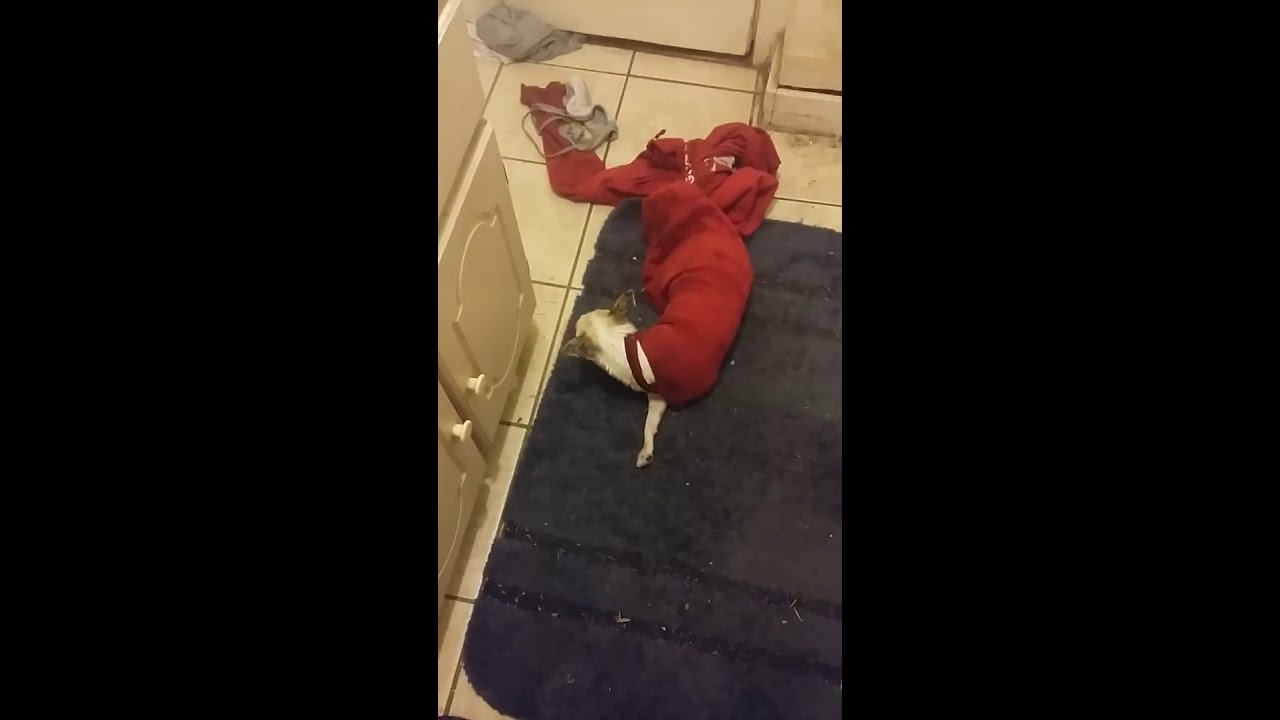The image captures a top-down view of a small toy dog, possibly a chihuahua, resting on a black mat placed over white square tiles. The dog is mostly wrapped in a red piece of clothing, resembling a sock or a sleeve, with only its head, neck, and one front left paw visible. The dog has a white body with black ears. To the left of the dog are white cabinets featuring small drawers with rose petal handles and etched square designs. The right and left edges of the frame are bordered by black backgrounds, covering about a third of the image. The setting appears well-lit, suggesting the shot was taken during the day.